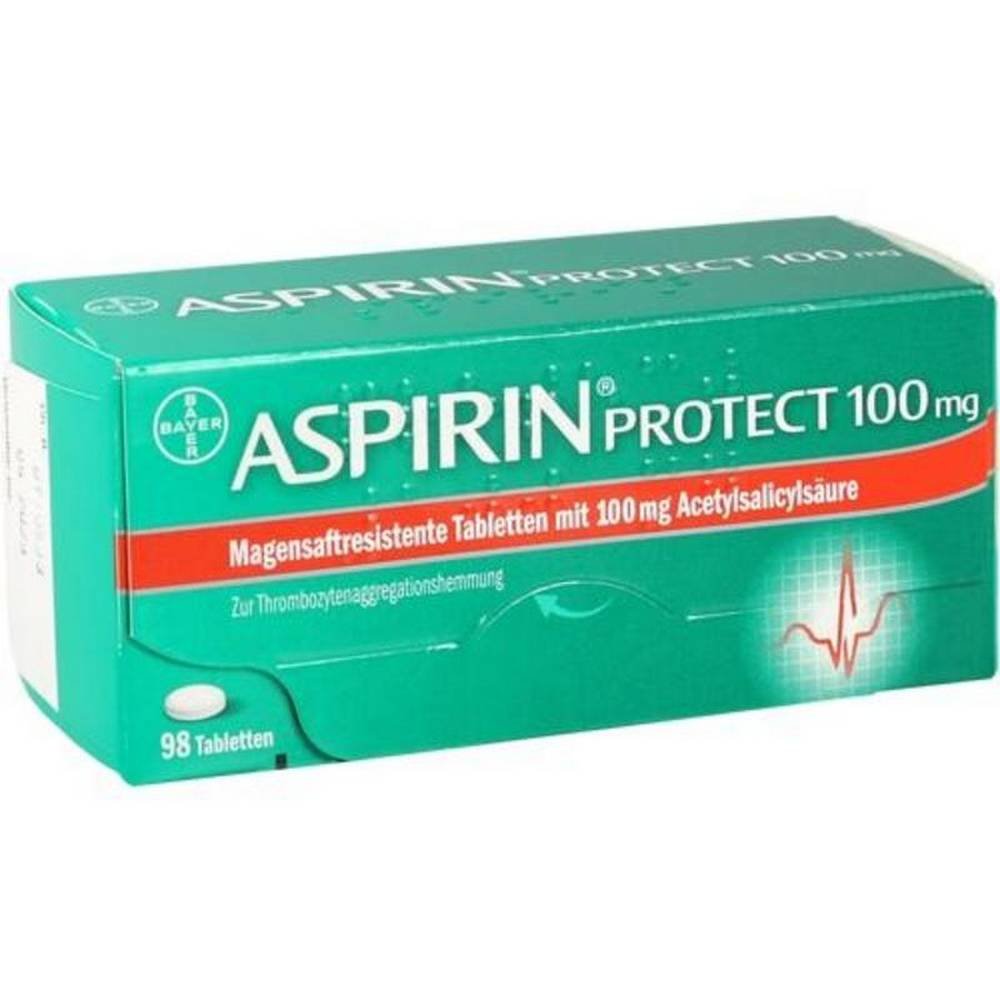This is a detailed photograph of a rectangular box of aspirin, predominantly aqua green in color. The box is positioned to show its top, front, and left side clearly, while the right side remains hidden. On the top of the box, the text reads "Aspirin Protect 100mg" in bold white font, alongside the Bayer brand symbol located in the top left corner.

The front of the box prominently features the Bayer logo, with "Aspirin" again displayed in large white letters, followed by "Protect 100mg." A distinctive red horizontal stripe runs across the center of the front face, bordered by white trim on both the top and bottom. Inside this red strip, in less readable text, it spells out "Magensaftresistente Tabletten Mit 100mg Acetylsalicylsäure." Beneath this, in very small white letters, there is additional text: "Zur Thromboseprophylaxe." 

In the bottom left corner of the box, there is an image of a single white tablet and the notation "98 Tabletten," indicating the quantity. The overall composition suggests a product image suitable for a retail website, showcasing the packaging details and brand information for consumer reference.